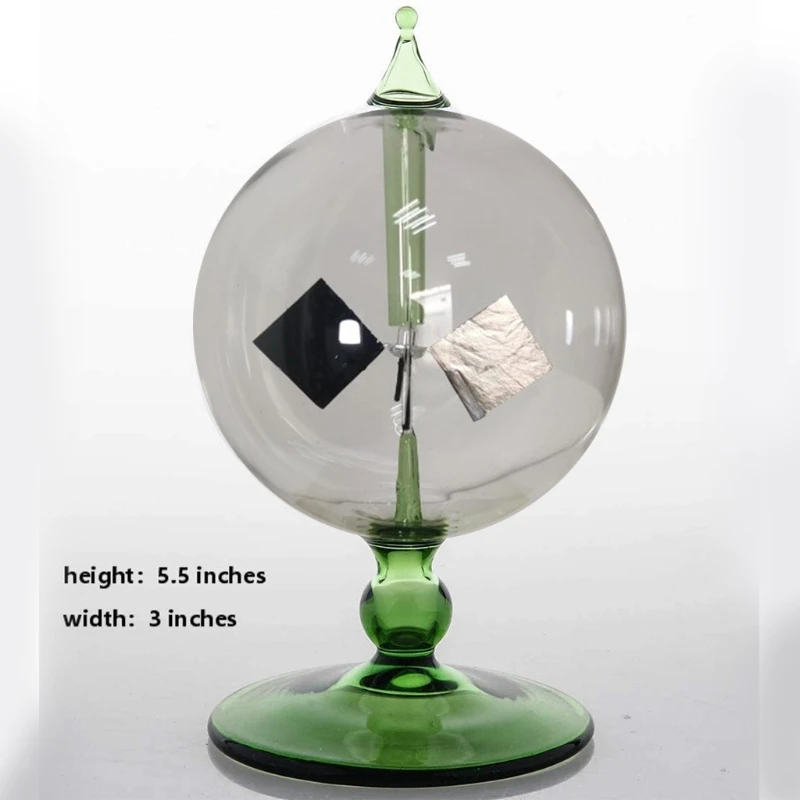In the image, there is a striking tabletop decor piece made entirely of glass, designed as a spherical orb measuring 5.5 inches in height and 3 inches in width. This glass sphere features a central column running vertically through its middle, which supports two diamond-shaped foils – one black and one silver – giving the item a balanced, dynamic look. At the top of the orb, there's a small green glass triangular element, adding a touch of color. The sphere is elegantly mounted on a glass base, reminiscent of a wine glass but with a rounded green ball forming the base instead of a tall stem. The base itself is also distinctly green. On the left side of the image, there are black letters on a white background indicating the dimensions: "height: 5.5 inches" and "width: 3 inches." The purpose of this intriguing object is unclear, but its aesthetic appeal is unmistakable.